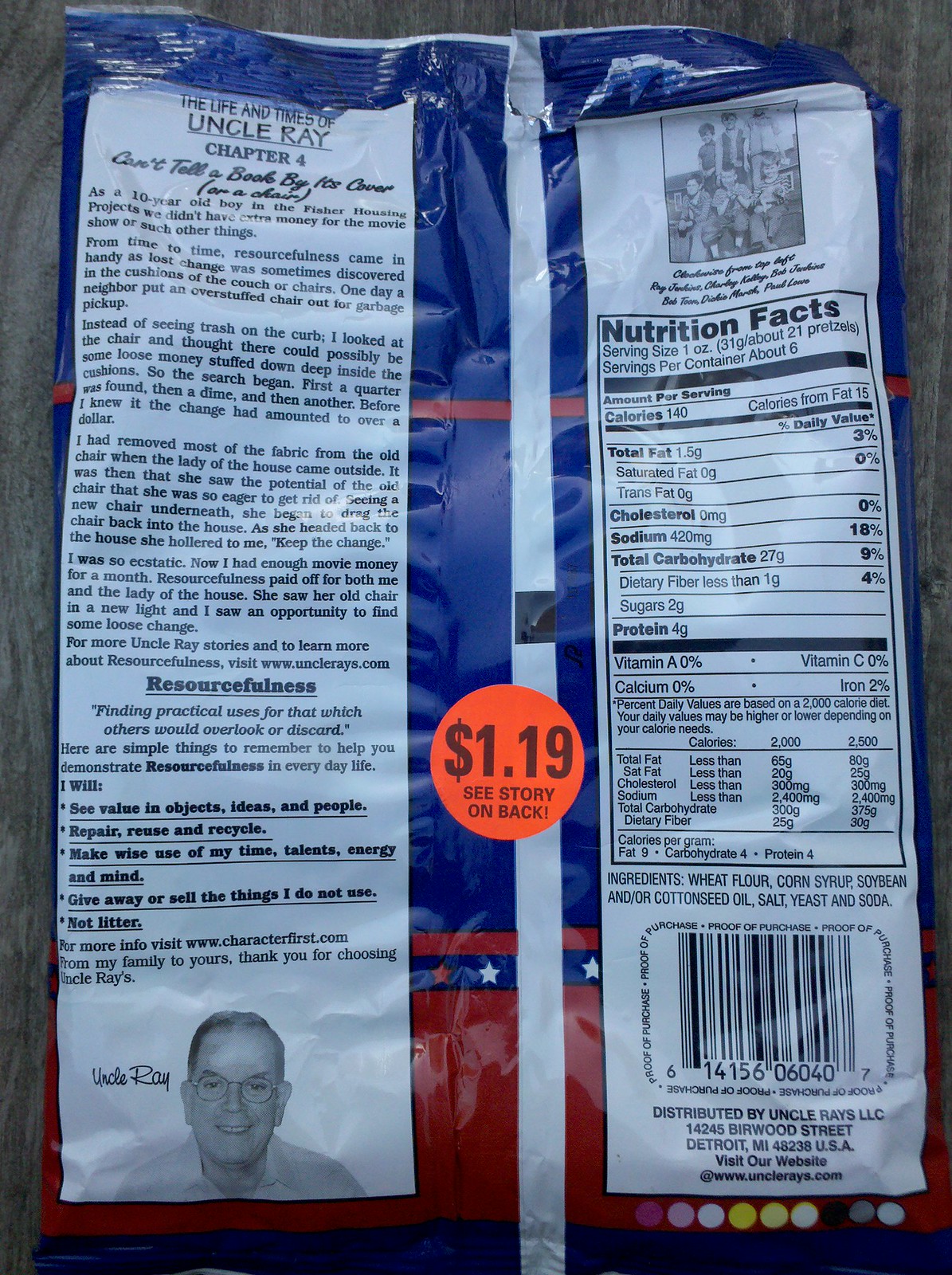This image showcases the back of a snack bag, placed on a gray wood grain surface. The bag is vividly designed, predominantly blue with red stripes, and features a line of red and white stars against a blue background at the bottom. Central to its design is an intriguing narrative titled, "The Life and Times of Uncle Ray, Chapter 4: Can't Tell a Book by Its Cover." This story detail accompanies extensive product information, including nutrition facts.

The packaging creatively arranges this information within white vertical rectangles, each one adorned with blue text. Prominently displayed is an illustration of an older man with glasses labeled "Uncle Ray," his signature elegantly inscribed next to the portrait. 

At the heart of the bag is a bright orange circular price sticker reading "$1.19," accompanied by the enticing prompt, "see story on back." Above the nutrition facts area, there is an image of a family, appearing to depict three boys and three girls, with some cursive writing adding a personal touch to the visual narrative.